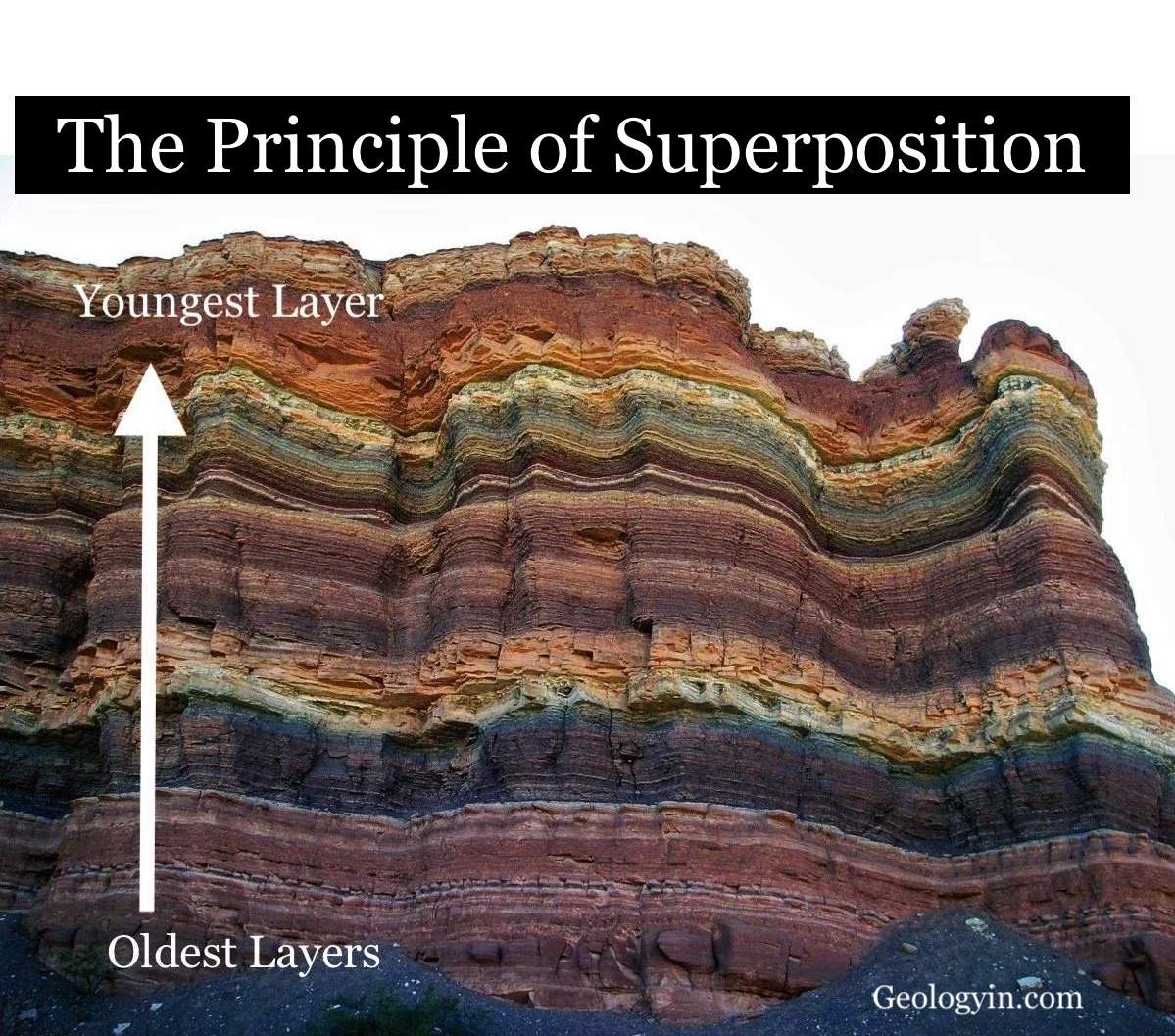The image illustrates the principle of superposition in geology, with the phrase "The Principle of Superposition" prominently displayed in white text on a black background at the top. Below, the image transitions to a white background showcasing a richly colored, multi-layered rock formation. An arrow extends from the bottom to the top of the formation, indicating the relative ages of the layers, with labels "oldest layer" at the bottom and "youngest layer" at the top, both in white text. The rock formation displays a sequence of color transitions, from darker purples, oranges, and browns at the bottom, through shades of dark purple and bluish tints, to thin strata of green, followed by yellows, oranges, and various shades of brown towards the top, culminating in a greenish tint and an orangish-red layer. In the bottom right corner, the text "geologyin.com" is printed in white, suggesting the source of the image.